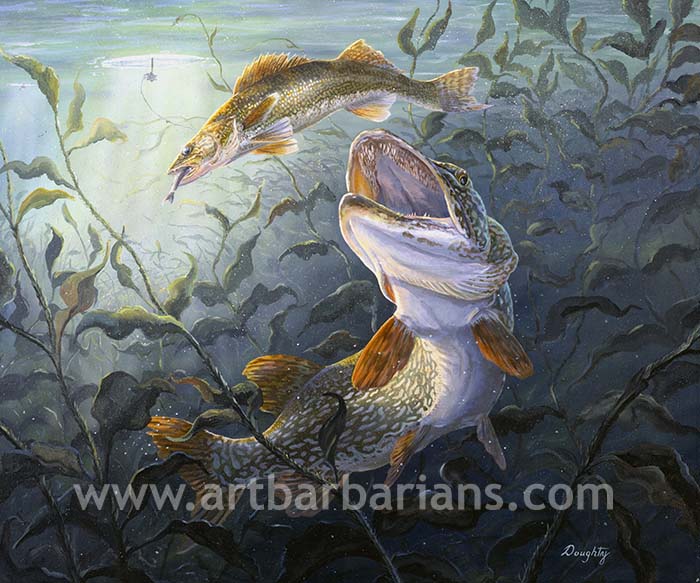The illustration depicts a murky freshwater underwater scene where a dramatic chain of predation unfolds. At the center of this scene, a hooked smaller fish has just caught an even tinier fish in its mouth. Below them, a much larger, menacing fish with an enormous mouth full of sharp teeth gazes upward, seemingly ready to devour the smaller, hooked fish. The background features seaweed and other aquatic vegetation, painted in hues of green and gray, adding to the murkiness of the water. A faint beam of light penetrates the water, illuminating the scene. The artist’s name, Dodie, is signed in cursive at the bottom right, and a website link, www.artbarbarians.com, is prominently displayed at the bottom of the picture.